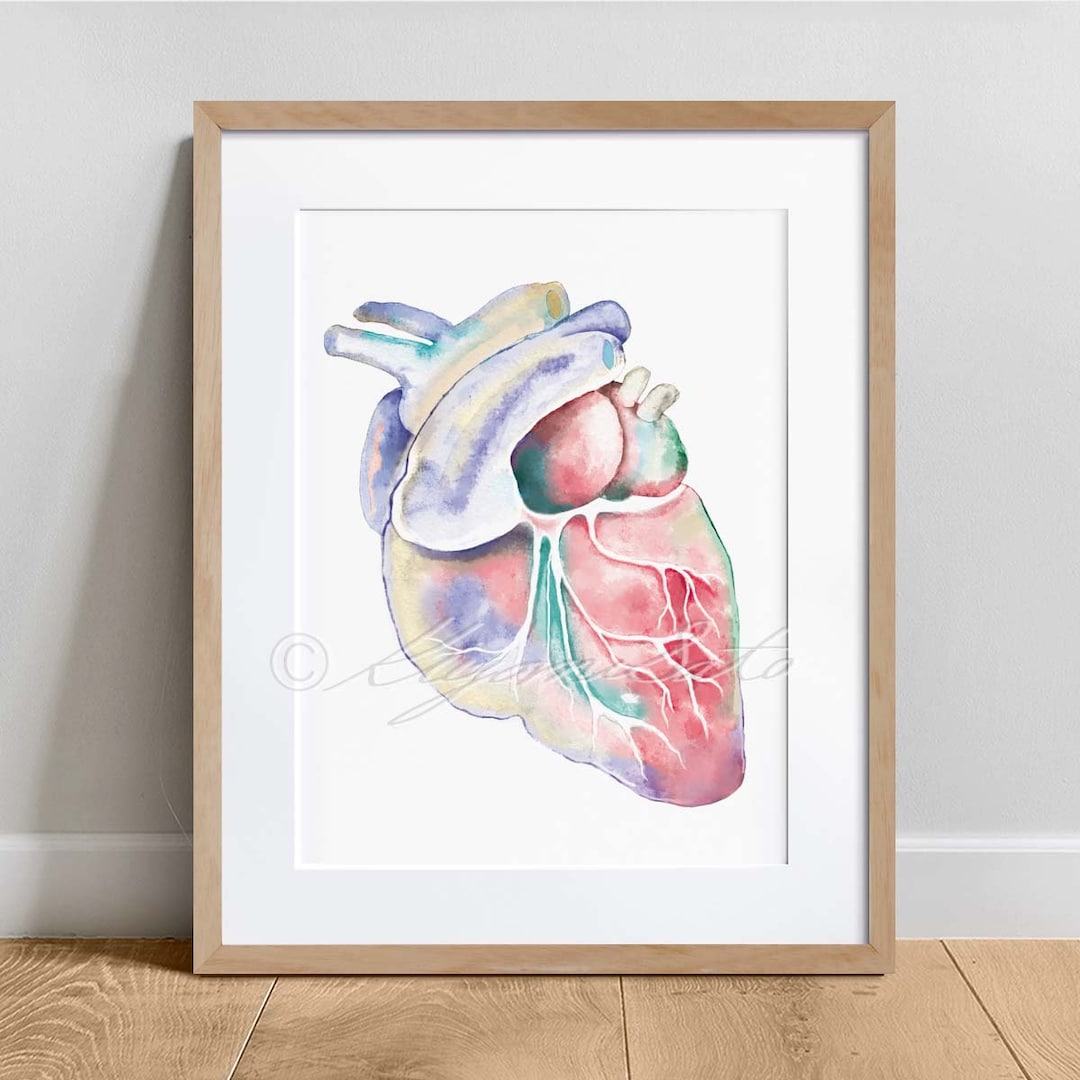This image depicts a photograph of a framed watercolor painting of a human heart, set against a white wall and on a light to medium brown wooden floor. The frame, which is a light brown color similar to the floor, leans against the wall and contains a white matting around the painting. The heart illustration within the frame is rich in detail, showcasing various anatomical features with hues of red, pink, green, blue, and purple. The ventricles and arteries are clearly visible, extending out from the heart, adding to the semi-realistic, yet artistic quality of the piece. A visible watermark overlays the entire image, bearing the copyright symbol followed by what appears to be the text "KAJOMILATO," likely identifying the brand or artist of the artwork.